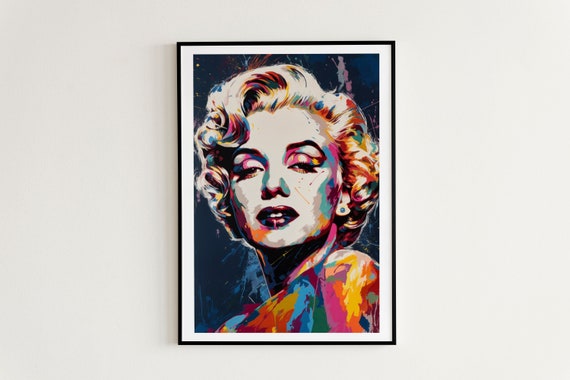This is an art print of Marilyn Monroe displayed on a white wall, encased in a slim black frame with a white border. The artwork features a headshot of Marilyn Monroe in a pop art style, recognizable by her distinctive makeup, hairstyle, and iconic red lips. Though her face remains predominantly white, it is accentuated by a vivid array of colors. Her hair features hues of orange, red, and blue, while her left shoulder and upper chest are splattered with a vibrant mix of rainbow colors, including pink, yellow, red, blue, green, and purple. The backdrop of the painting is a dark, navy blue, which contrasts sharply with the colorful splashes that envelope the lower part of her image. The piece is an abstract and colorful rendition of Monroe, preserving her likeness while adding an artistic twist with its myriad of paint splatters. The entire composition, set within a vertical rectangular format, is likely at least 9 by 13 inches or larger.